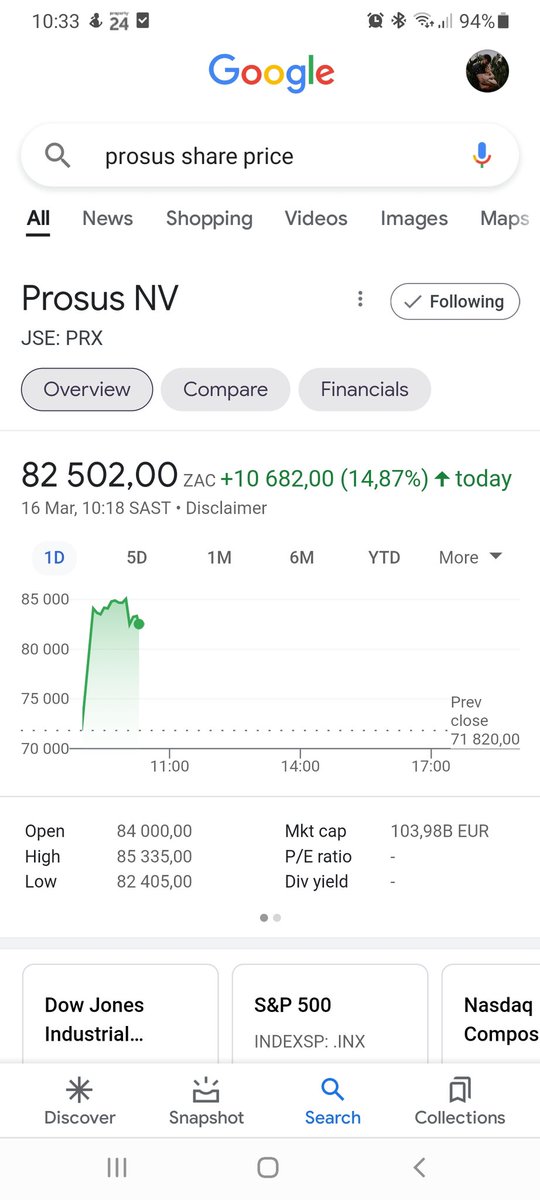A person checked the current share price of Process NV and saw a detailed overview. The share price is listed as 82,502 ZAC, with a notation of "+10,682 ZAC," indicating a 14.87% increase today. The market appears to still be open, but the exact time of the day is unspecified. A graph displays significant trading activity, especially before 11 AM. The stock opened at 84,000 ZAC, reached a high of 85,335 ZAC, and dipped to a low of 82,405 ZAC. The specific index, whether Dow Jones or S&P, wasn't clearly indicated.